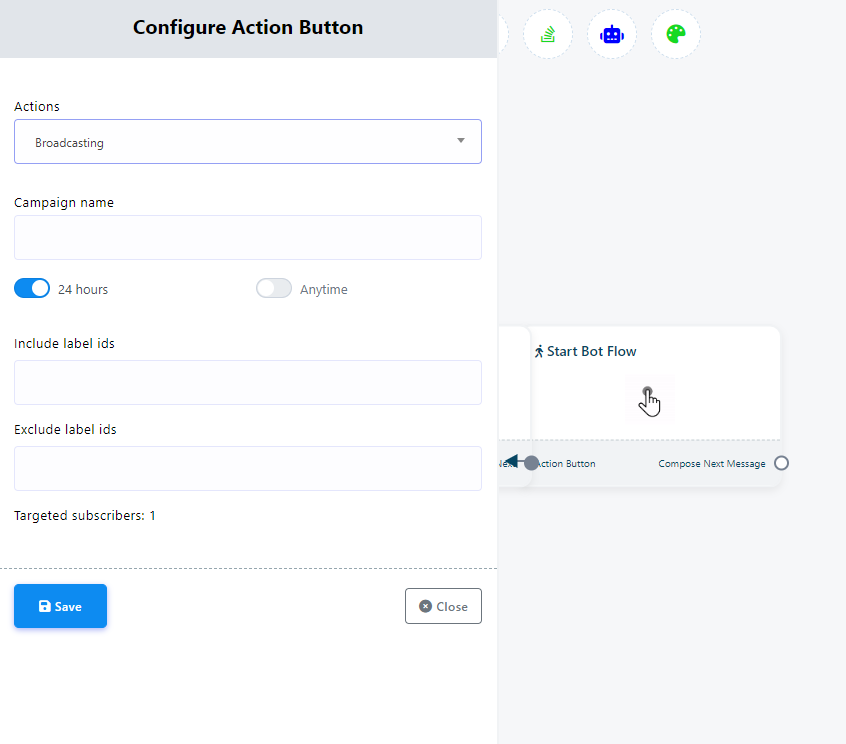This image appears to be a screenshot of a configuration page for setting up actions related to broadcasting for a bot. On the left-hand side of the screenshot, there is a prominent pop-up window with various settings.

At the top of the pop-up, a heading reads "Configure Action Button Actions: Broadcasting." Below this, there is a text box labeled "Name" which is currently blank. The section below has two radio buttons; "24 hours" is selected, and "Anytime" is unselected. 

Further down, there are two sections for managing label IDs: "Include Label IDs" and "Exclude Label IDs," both of which contain drop-down boxes that are currently empty.

Additionally, there is a numerical field labeled "Target Subscribers," which is set to "1." At the bottom of the pop-up on the left side is a blue button labeled "Save," and fittingly, on the right side, there is a white button labeled "Close."

The part of the page that the pop-up obscures shows a series of icons at the top. The first icon is unidentified, the middle icon is a blue robot, and the last icon is a green paint easel, likely for theme or color selection. Below these icons, there is a visible text box that reads "Start Bot Flow," indicating that this configuration pertains to bot flow actions. There are also options for "Action Button," which triggered the pop-up window, and "Compose Next Message," which remains unselected.

This detailed screenshot suggests the user is in the process of configuring broadcasting actions for a bot, specifying parameters like time settings, label IDs, and target subscribers, while navigating a user interface with various customizable icons and settings.